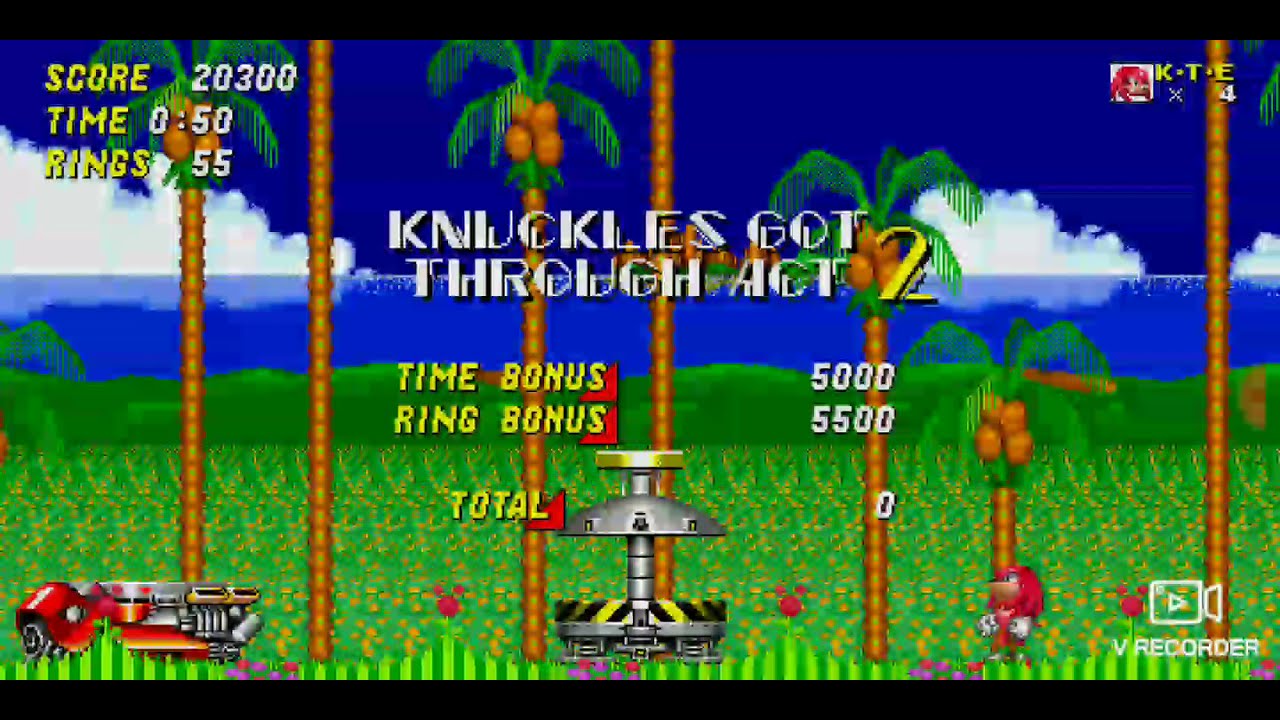The screenshot from the Sonic the Hedgehog video game depicts the pause menu screen featuring the character Knuckles, a red echidna with long red hair. Prominently in the center, white text declares, "Knuckles got through Act 2," alongside a time bonus of 5,000 points and a ring bonus of 5,500 points. The top left corner displays the player's score of 20,300 points, a time of 0 hours and 50 minutes, and a ring count of 55. The background showcases a vibrant scene with a field of green grass studded with palm trees bearing coconuts, under a blue sky. In the center, there's a metallic, jumping mechanic robot, and to the left, part of another robotic structure is visible. This detailed snapshot encapsulates the game's dynamic and colorful environment.